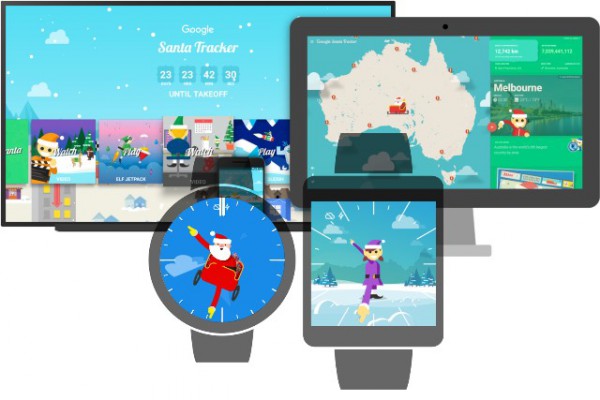In the image, there are multiple screens displaying Christmas-themed visuals. On the left, a large screen, likely a monitor or television, features a variety of cartoony Christmas images. Prominently displayed in the center of this screen is an app titled "Santa Tracker," set against a snowy blue sky with a countdown indicating the time until Santa's takeoff. This app appears to be designed for children. 

Adjacent to this, on the right, is a tablet displaying the same "Santa Tracker" app. Below this setup, there's a digital illustration of a watch that features Santa Claus, with his arms serving as the watch hands. To its right, another screen shows a smartwatch displaying an elf, whose arms are also ingeniously used as the watch hands.